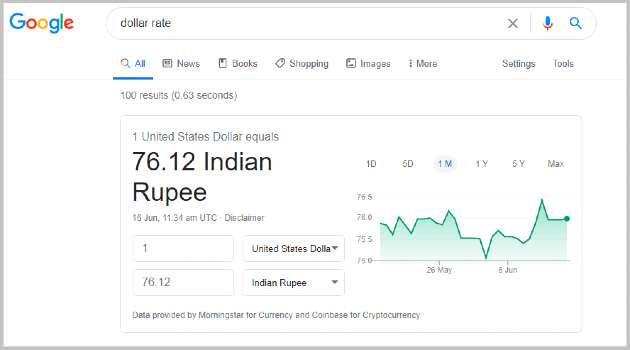The image depicts a Google search results page with a thin gray border around its perimeter. In the top-left corner is the Google logo, featuring the classic primary colors: a blue capital 'G,' followed by a red 'o,' yellow 'o,' blue 'g,' green 'l,' and a red 'e'. 

Below the logo, the search bar displays the query "dollar rate," accompanied by an 'X' for clearing the text, a microphone icon for voice search, and a magnifying glass icon for executing the search. 

Underneath the search bar, a navigation strip appears with a rainbow-colored magnifying glass icon next to "All" in blue, underlined text. The navigation options include "News," "Books," "Shopping," "Images," and a "More" option denoted by three vertically stacked dots. To the far right of the navigation strip, "Settings" and "Tools" are listed.

Further down, the page indicates "About 100 results" generated in "0.63 seconds." The first search result states: "1 United States Dollar equals 76.12 Indian Rupee" with a timestamp of "15 June, 11:34 AM UTC," followed by a disclaimer. A rectangle next to this result indicates it is the top result.

This section is followed by more detailed information: "1 United States Dollar" with a drop-down menu and "Indian Rupee" also with a drop-down menu. Below that, a green graph illustrates the exchange rate trend. At the bottom, there is a note stating, "Data provided by Morningstar for Currency and Coinbase for Cryptocurrency."